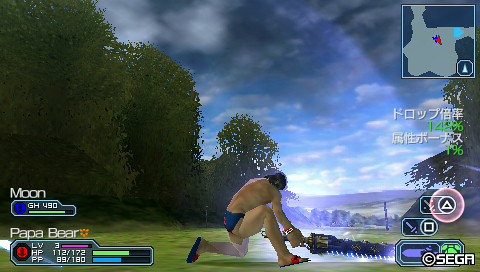This is a detailed screenshot from a Sega video game. In the bottom right corner, the Sega logo is visible, confirming the game's developer. The user interface on the left side of the screen displays several player stats. At the top, an icon representing the player character is visible, accompanied by various status bars. The first bar, labeled "LV," which likely stands for "Level" or "Lives," shows a value of three. Below it, a purple "HP" bar indicates the character's health points, displayed alongside numerical values. Underneath the HP bar, a green bar, filled to about two-thirds capacity, is present without an explicitly visible label. Additionally, a blue "PP" bar tracks another game metric, possibly "Power Points" or a similar attribute.

In the center of the screen, the main character is depicted. He is a man with dark hair, attired only in shorts, and he is crouching. The character wields a glowing blue sword, which he is holding on the ground, illuminating a small area around it. The setting is a picturesque field, with trees dotting the landscape on the left side and a partly cloudy blue sky stretching across the background.